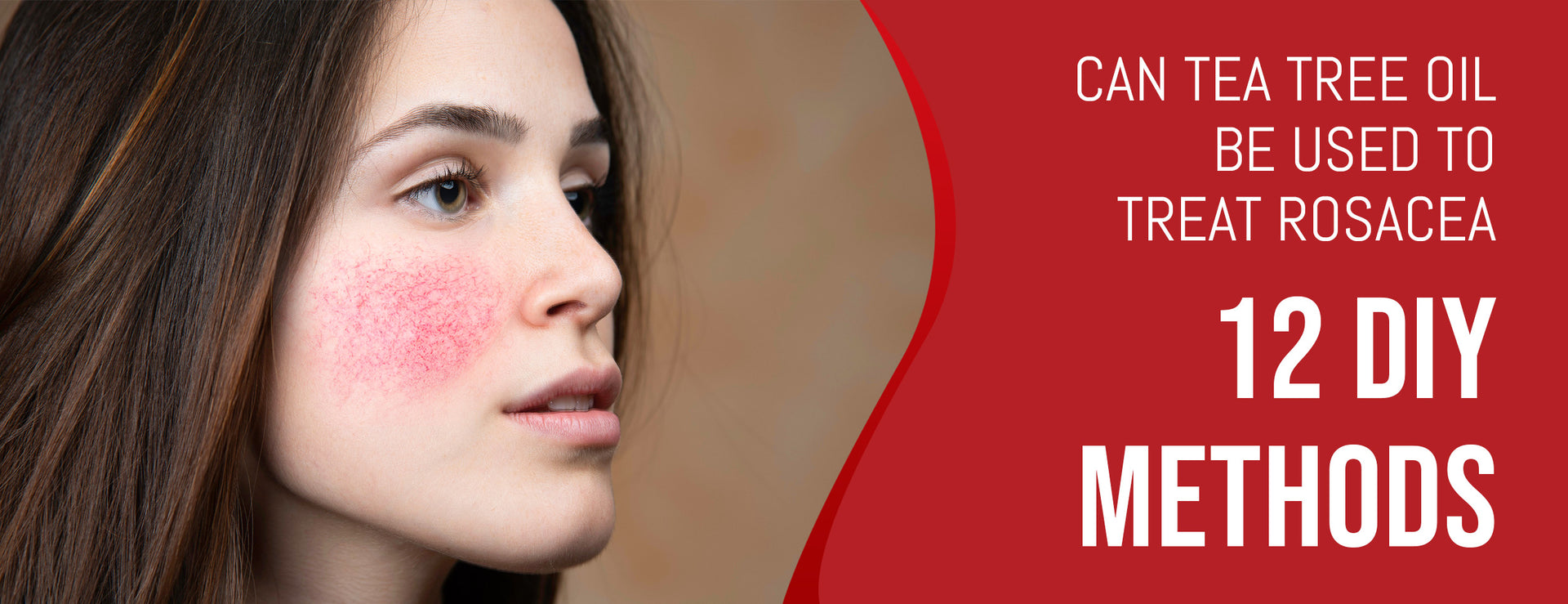The advertisement features a striking, long, and narrow widescreen image. On the left, a young woman, possibly in her late teens to early 20s, with long brunette hair and greenish-brown or hazel eyes, gazes to the right. Her complexion is fair, indicating she might be Caucasian or Latino. Her right cheek prominently displays small, red, splotchy bumps indicative of rosacea against a brown background. Her expression is neutral, with slightly parted lips.

On the right side of the advertisement, separated by a swooping line, a bold red background showcases text in all caps: "CAN TEA TREE OIL BE USED TO TREAT ROSACEA?" Directly below, in white and still bold, it reads "12 DIY METHODS," suggesting an article header or blog post link. The text and graphics are organically integrated, emphasizing a natural solution for the skin condition depicted.